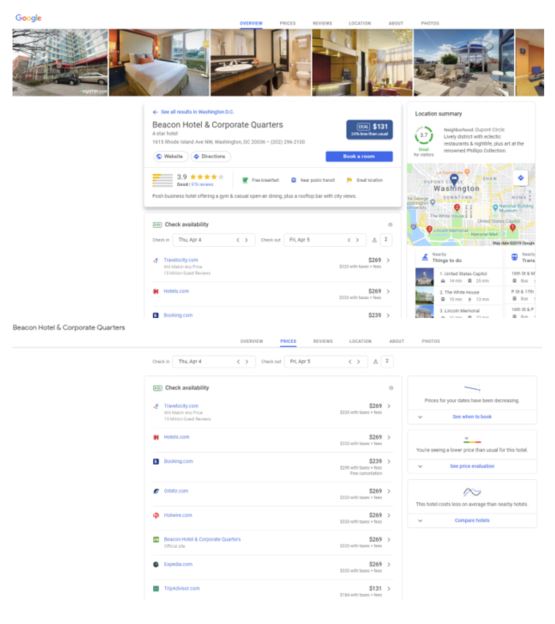The image depicts a Google search results page on a computer screen, specifically featuring details about the "Beacon Hotel and Corporate Quarters." In the upper left corner, the familiar Google logo is prominently displayed in its signature rainbow colors. Below the logo, a horizontal strip of five and a half rectangles showcases vibrant photos of hotel interiors and exteriors.

At the top of the page, the "Overview" tab is selected, which displays comprehensive information about the featured hotel. Beneath the colorful photos, a highlighted section provides essential details about the Beacon Hotel and Corporate Quarters, including a "Check Availability" option. This option lists various booking platforms, such as hotels.com and booking.com, along with their respective price offerings.

Further down the page, additional "Check Availability" buttons accompanied by prices from different sites are visible, offering more options for potential bookings. On the right side of the screen, there is a map of Washington, D.C., featuring a prominent blue marker indicating the location of the Beacon Hotel. Surrounding this are several smaller red markers pointing out other nearby establishments. The entire page is set against a clean white background, with the text primarily in black and occasional elements in blue.